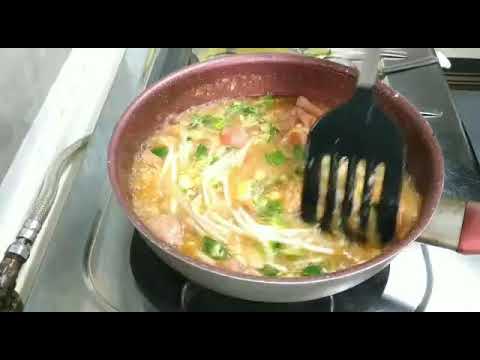This rectangular image, approximately three inches wide and two inches high with thin black borders at the top and bottom, presents a top-down view of a culinary scene set in a kitchen, most likely inside a restaurant. Dominating the center of the image is a large metal pan, with a shiny aluminum or steel exterior and a light gray interior, sitting on a stainless steel gas stovetop. A black spatula extends from the top of the image, actively stirring what appears to be a partially-cooked dish. The contents of the pan include long white noodles, small bits of grain, meat chunks, onions, and a runny egg mixture, suggesting the preparation of an omelet or ramen soup. The overall color palette includes black, gray, white, tan, orange, pink, green, red, and brownish-orange hues. Additionally, the image features another bowl on a separate burner visible at the top of the screen coming in from the lower left-hand corner. This comprehensive scene highlights the dynamic and detailed process of meal preparation in a professional kitchen environment.